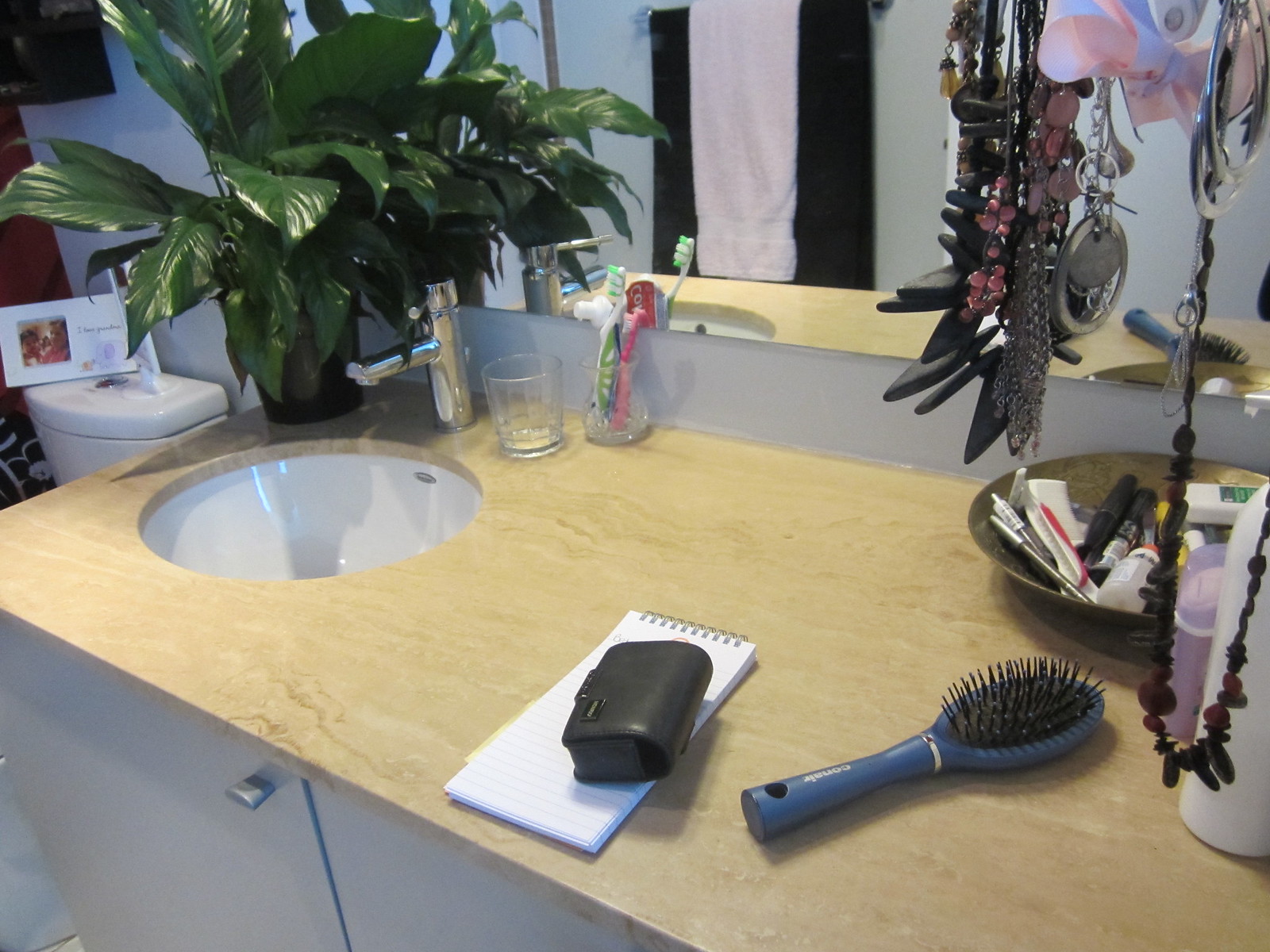This color photograph encapsulates a detailed scene of a bathroom counter with a brown surface. On the far left, a small circular sink basin is featured with a single-handle faucet for temperature control. Adjacent to the faucet on the right is a small empty drinking glass, followed by another glass containing two toothbrushes—one green and one pink—and a tube of Colgate toothpaste.

Moving further along the counter, a white spiral notebook is seen with a black case resting on top. A Conair paddle-style hairbrush with a blue handle is positioned next to a dish filled with various miscellaneous items. Among these items is a stick deodorant in a purple container and a tall white bottle.

At the top right corner of the counter, numerous necklaces dangle, hanging from an unidentified item. Above the counter is a mirror reflecting a towel rod that holds two black towels with a white towel draped over them. The far-left edge of the image reveals the top of a toilet tank, which has a greeting card propped up on it. Nestled to the left side of the faucet is a potted plant boasting shiny dark green leaves, adding a touch of nature to the scene.